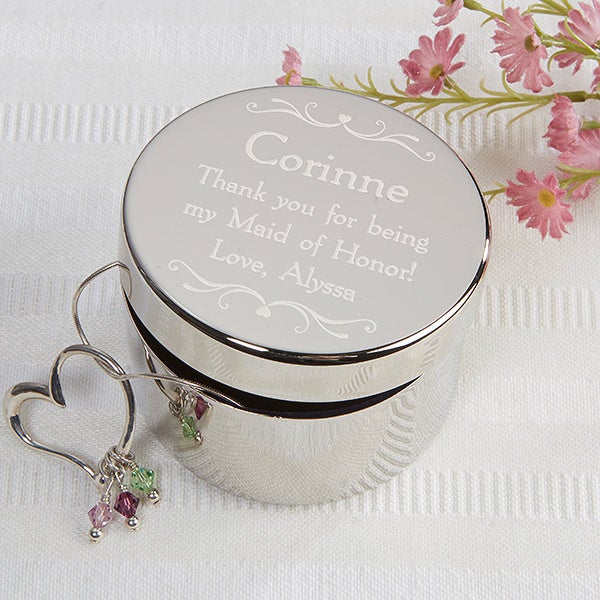This color photograph, captured in a square format with a top-down perspective, features a shiny, silver cylindrical trinket box. The lid of the trinket box, which is slightly lifted, reveals a silver wire emerging from inside. This wire runs through a heart-shaped metal ring, which is adorned with three dangling jewels suspended from delicate chains: a green jewel on the right, a deep purple jewel in the center, and a light pink jewel on the left.

The lid of the trinket box is inscribed in white text that reads, "Corinne, thank you for being my maid of honor. Love, Elisa." The text is flanked by wavy patterns of hearts above and below, adding to its decorative appeal. The trinket box rests on a white, textured tablecloth that is embroidered with pink flowers along green stems, particularly notable in the top right corner of the photograph. This setting creates a graceful and elegant composition, characteristic of Photographic Representationalism and Product Photography.